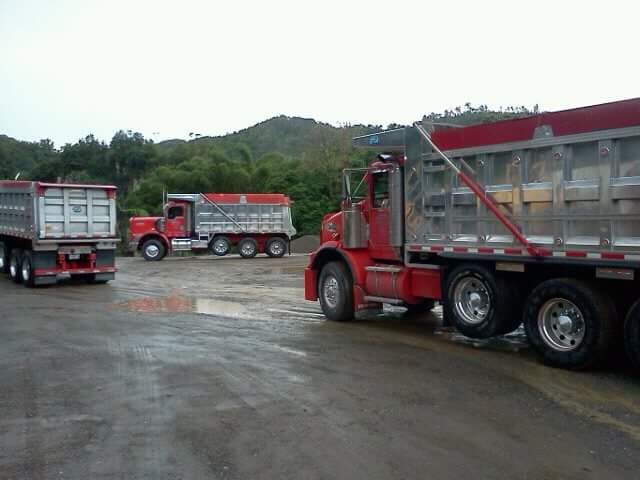This horizontal, color photograph, taken outdoors during the day, showcases a slightly overcast sky with hints of blue peeking through the clouds. In the background, lush, vibrant green trees, bushes, and a grassy hill contribute to the scenic, natural setting. The foreground is dominated by a damp, dark gray paved lot, interspersed with small puddles reflecting the wet surface.

The main subjects of the photograph are three red and silver dump trucks, each prominently featured at different positions within the frame. On the left, only the back of the first truck is visible with its stainless steel dump bed and part of its black and silver wheels. The middle truck, positioned farther away, reveals its full side profile, highlighting its red cab and roof, along with the metallic sheen of its cargo area. The third truck, situated to the right and closest to the camera, presents a frontal view that emphasizes its red cab and the consistent design shared among all three trucks, including the black, silver-trimmed tires and stainless steel dump compartments.

The image is devoid of people and buildings, focusing purely on the trucks and their surroundings, emphasizing the industrial yet tranquil outdoor setting.